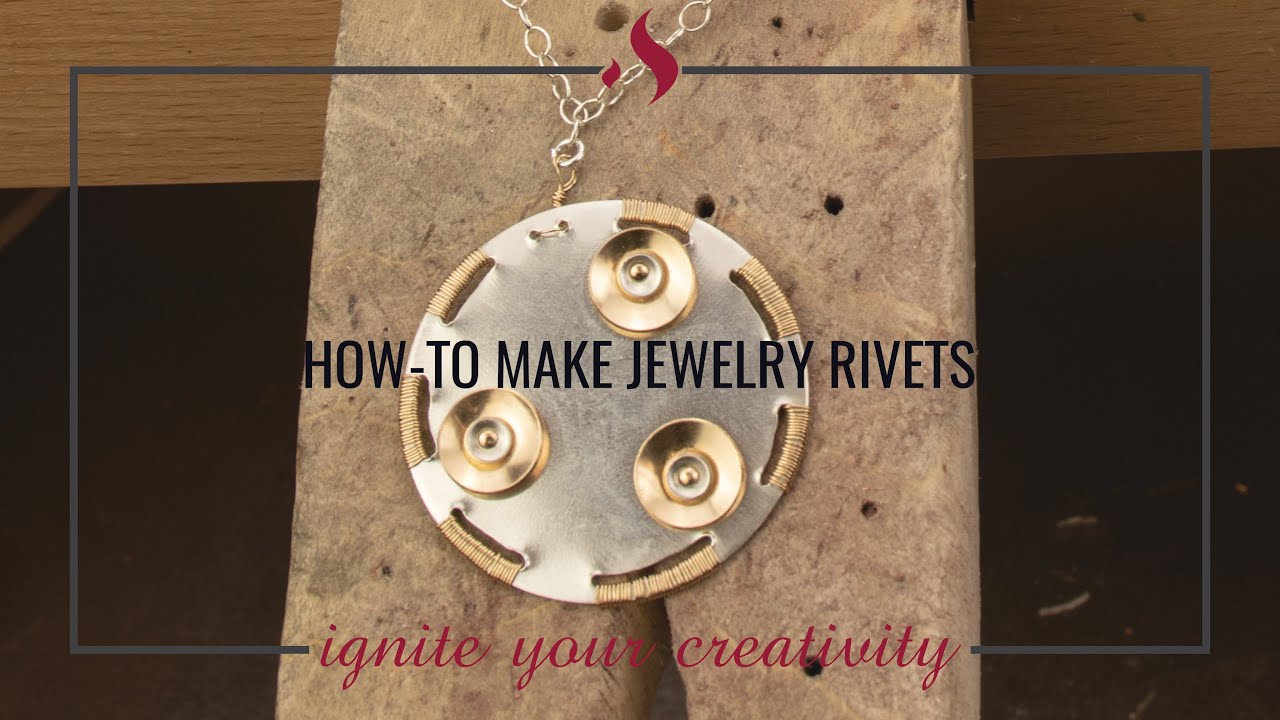The image is a detailed title card for a jewelry-making tutorial titled "How to Make Jewelry Rivets," presented in a black Arial Narrow font. The design features a gray rectangular border, interrupted at the top by a small cartoon flame illustration with red squiggly lines and at the bottom by the text "Ignite Your Creativity" in the same red color. Central to the image is a close-up of a circular metal pendant, displaying intricate craftsmanship. The pendant, appearing silver, is adorned with what looks like gold, brass, or bronze wire intricately woven into slots on its surface, along with three gold rivets. The pendant is attached to a silver chain, both resting on what seems to be a wooden or stone block, enhancing the rustic and artisanal appeal of the piece. The overall composition effectively combines text and imagery to convey a creative and instructional theme.